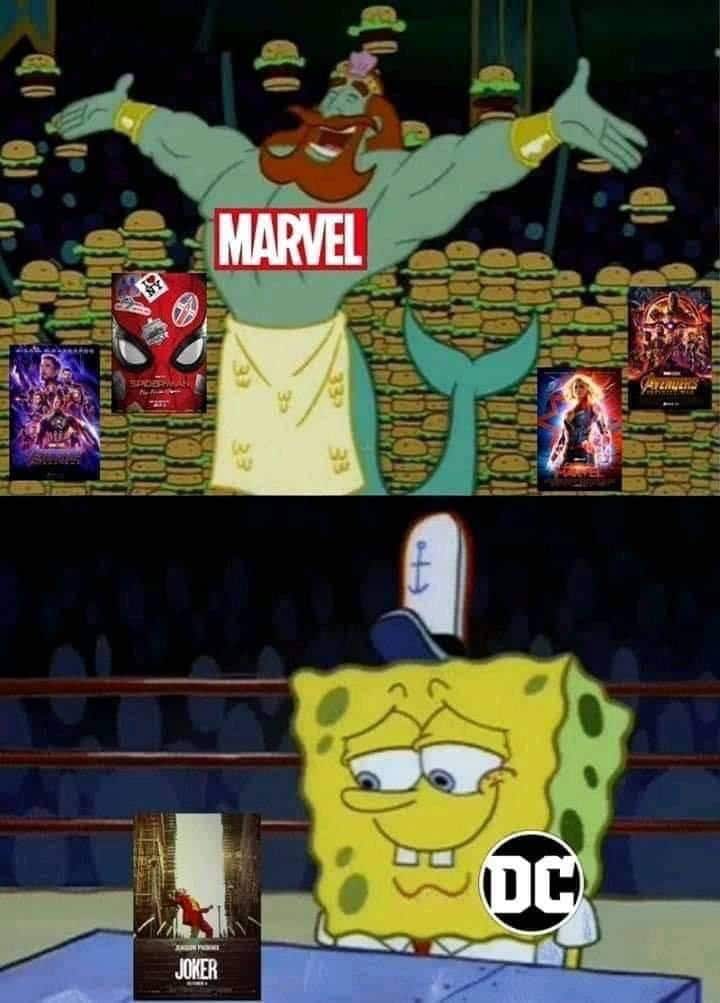The meme features a two-panel layout with superimposed logos and images. 

In the top panel, there's a screenshot from a SpongeBob SquarePants episode. The background depicts a dark blue, open expanse of water. Descending from behind the central figure is a towering stack of Krabby Patties, with additional patties floating down to join the stack. The central figure is a muscular mermaid adorned with a yellow apron, a long red beard, and a crown. This figure is labeled "Marvel." Superimposed on the stack of Krabby Patties are screenshots of various movie posters, including Spider-Man, The Avengers, Captain Marvel, and another Avengers film.

In the bottom panel, SpongeBob is depicted in what appears to be a wrestling ring, complete with numerous circular shapes in the background representing people's faces. He sits in front of a counter, gazing longingly or lovingly at it. SpongeBob is wearing his work hat and is labeled "DC." The area he is staring at features a superimposed screenshot of the Joker movie cover.

The meme juxtaposes the prolific and celebrated Marvel Cinematic Universe (represented by the muscular mermaid and abundant Krabby Patties) with DC's focused admiration for its film, Joker (represented by SpongeBob's longing gaze).